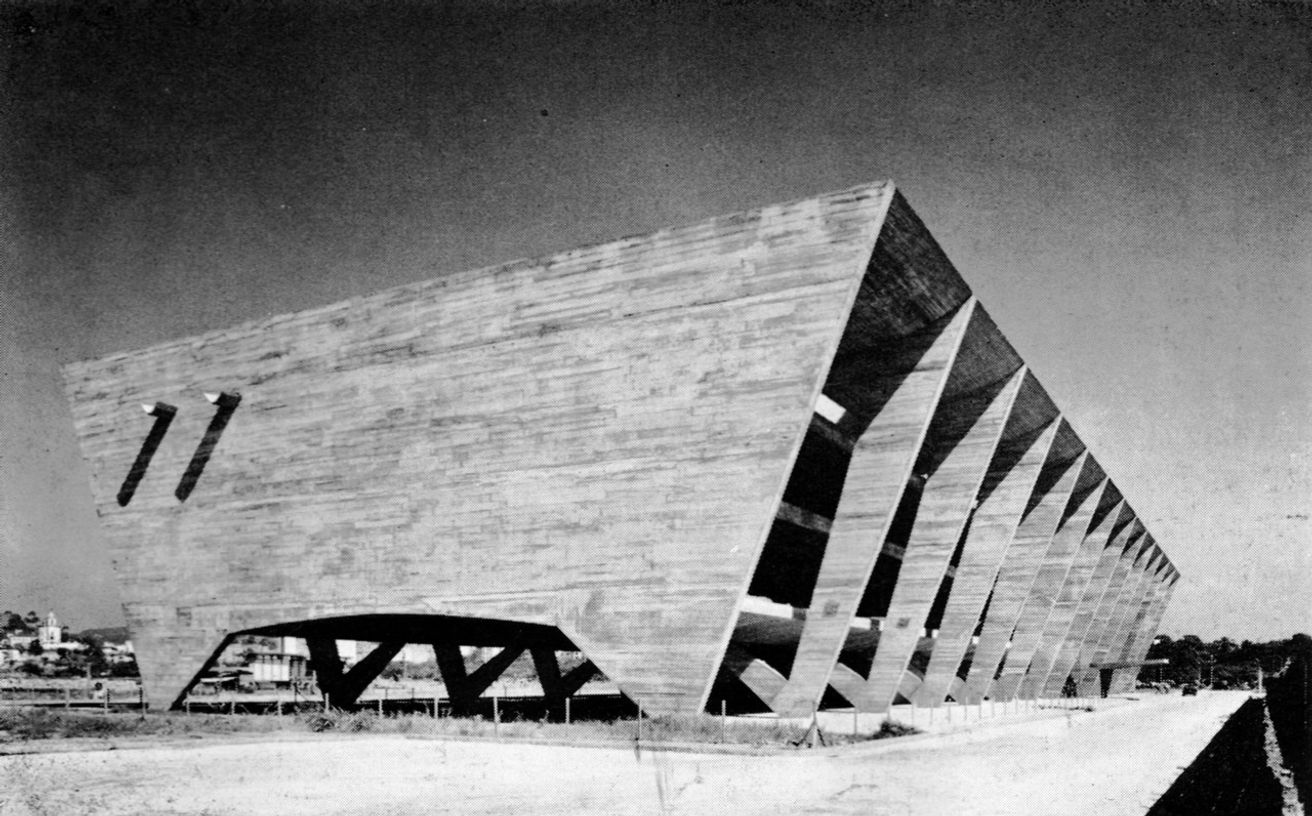This black-and-white photograph captures a peculiar, architecturally artistic structure set against a dark upper left sky that gradually lightens towards the lower right. The focus of the image is a large, elevated structure resembling a giant coffee table, boasting multiple levels—at least three—with a flat top and flat sides. The structure's lower portion features triangular, fang-like feet, and there is a raised opening that seems to serve as an entrance on the right-hand side. The right side of the structure is divided into at least ten sections by tall, vertical gray boards or flat columns supporting the flat-looking roof. Two wooden pegs protrude from the upper left corner of the structure, adding to its unusual appearance. The grainy texture of the photograph suggests an old, possibly historic image. The landscape around it appears flat, potentially dirt, and there's a heavily shadowed area or a road on the lower right. Background details include more conventional buildings visible in the distance on the left side.